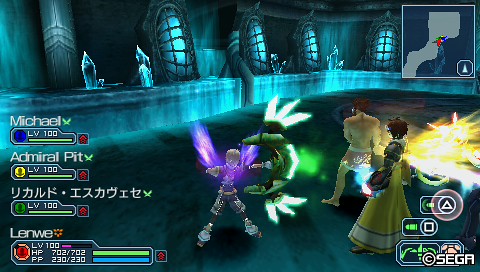In this detailed screenshot from a video game, we can observe four distinct characters actively engaged in what appears to be a battle. Their names, listed on the left-hand side of the screen, include Michael, Admiral Pitt, a third character with a name in Japanese characters, and Lenwee. All characters are at level 100. Michael and Admiral Pitt have light green bars indicating full health, whereas Lenwee has a purple health bar that is only 30% filled. Each character's status includes an LV100 notation and accompanying symbols in different colors—green, yellow, and red respectively—alongside measurements for HP (702/702) and PP (230/230).

The setting of the game is a dark, fantastical cave-like structure adorned with luminescent turquoise crystals and columns. The characters are depicted with futuristic elements—one with purple wings, another emits a green light, one dressed only in shorts, and a figure in a yellow dress casting a yellow beam of light. The arena floor and upper levels are primarily blue, enhancing the futuristic and fantasy aesthetic.

Overlaying the gameplay is a small locator map situated in the top right corner of the screen, providing navigational assistance. Additionally, there's an overlay of the SEGA logo in white text at the bottom right, indicating it was added post-capture. This attachment partially obscures the in-game infographic. Overall, the vibrant battleground, detailed character stats, and mix of sci-fi and magical elements suggest a deeply immersive and dynamic gaming experience.